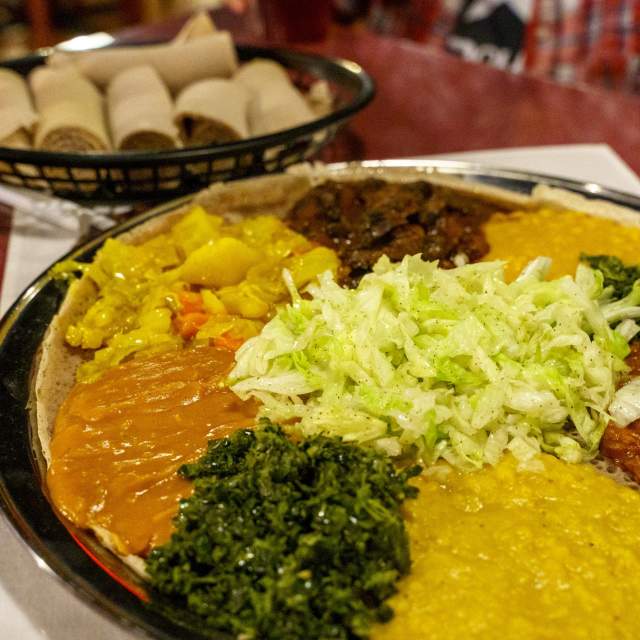The image features a square-format, color photograph showing a close-up of a round, silver-rimmed plate filled with various foods, viewed slightly from above. At the very bottom of the plate, there is a serving of dark green spinach. Moving clockwise, the next food item appears golden yellow, possibly applesauce or corn. Directly to the left of this is an orange-toned substance, which looks like gravy over a piece of meat. 

In the center of the plate, there is a pile of green shredded lettuce or cabbage, sprinkled with pepper for seasoning. On the upper left side lies some shell noodles, akin to macaroni and cheese. Adjacent to this, at the top, is a portion of brown meat accompanied by another yellow sauce. In the background, towards the upper left corner, there is a black round basket containing rolled-up tortillas or pastries with some brown filling visible.

The plate sits atop a white placemat, and the overall photographic style is realistic and detailed. The entire composition is rich with colors like green, yellow, orange, brown, tan, beige, and silver, emphasizing the varied food elements arranged radially around the central lettuce pile. The setting suggests the plate is on a table, though it's unclear whether the photo was taken indoors or outdoors or during the daytime or nighttime.